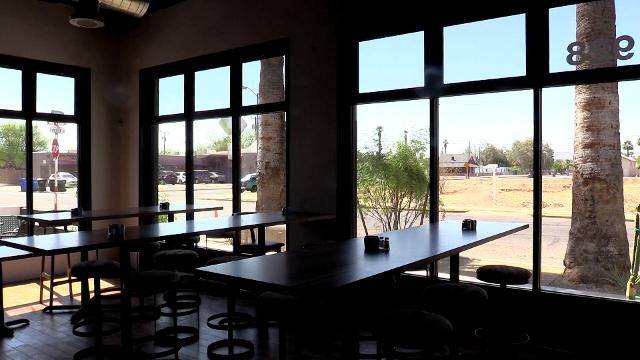This detailed photograph, likely taken inside a well-known Mexican restaurant such as Gallo Blanco, showcases an empty and serene setting. The image is captured from a corner perspective, revealing a series of long, light brown tables with stools instead of chairs, indicating a casual dining or bar-like atmosphere. Three tables are positioned towards the left and center of the restaurant, aligned with large panes of glass that allow a clear view of the outside.

The restaurant features a brick floor and a ceiling that hovers above the seating area. On the tables, only a few items like napkin dispensers can be seen, and there’s no food present, emphasizing the clean and tidy environment. Through the glass panes, the outdoor scene reveals a mix of elements including vibrant greenery, a couple of trees near the right side, cars, and other buildings across a parking lot and road. A stop sign can also be spotted, adding to the bustling yet rustic feel of the surroundings. The sky appears to be a bright blue, enhancing the contrast with the various colors inside the restaurant such as greens, black, gray, red, and blue.